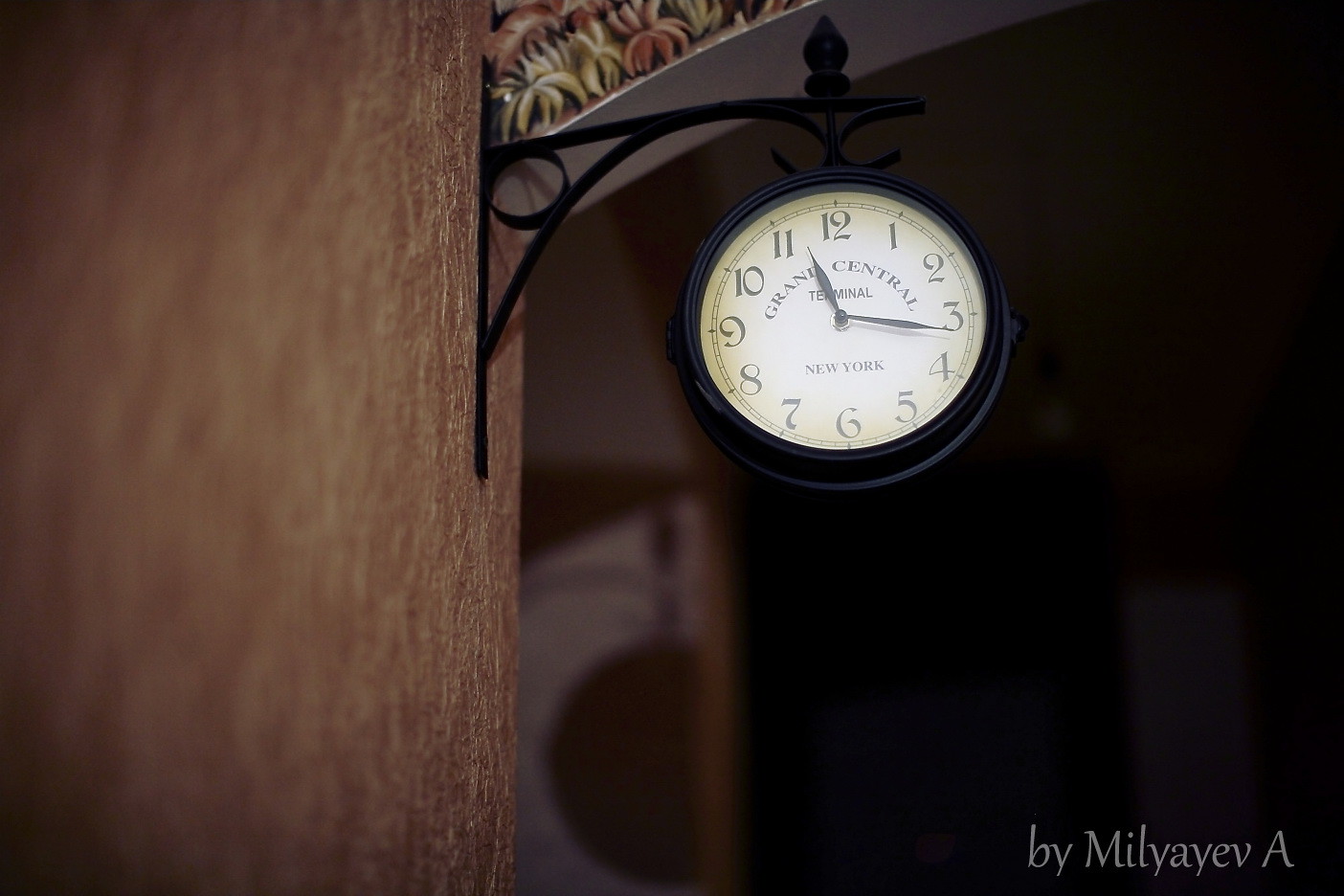In this detailed photograph, a vintage-style clock hangs from an ornate black wrought iron bracket, securely fastened to a wooden-styled wall. The clock has a black rim and an ivory white face, with black arms and numerals. The outer edge of the clock face carries a yellowish tint, adding to its antique appearance. The time shown is approximately 11:13. The clock prominently features the text "Grand Central Terminal" across its center, with "New York" just above the 6 o'clock position. Above the clock, the photo includes some indistinct, multicolored objects that resemble crustaceans. The background transitions from a wood grain texture on the left to a darker area on the right, possibly indicative of a doorframe. The image is credited to Milyaev A, as noted at the bottom of the photo, though some parts of the image remain slightly blurry.